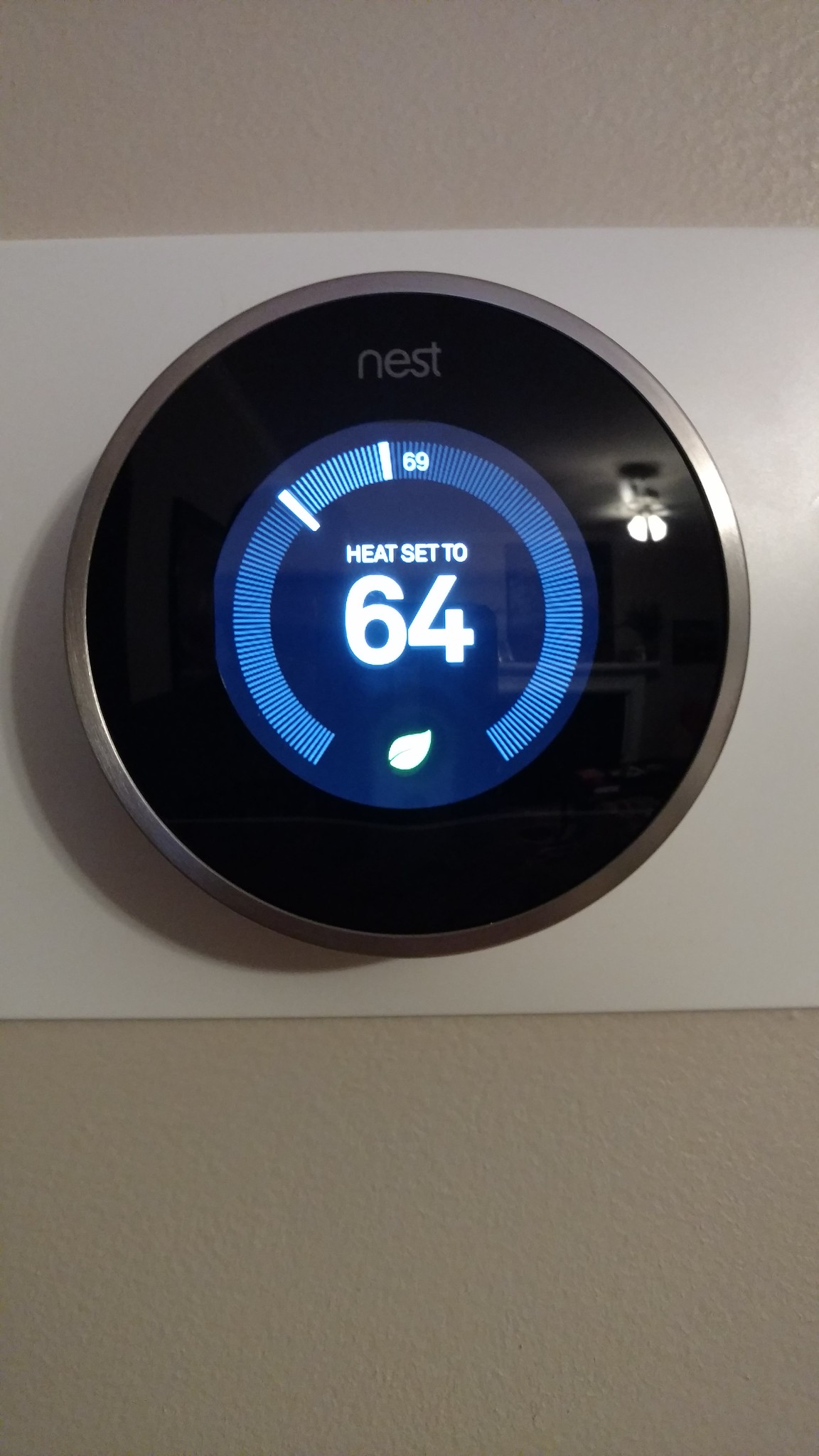This close-up photograph features a Nest brand thermostat, prominently showcased on a beige wall. The thermostat itself is strikingly circular, reminiscent of a stove dial with its substantial thickness suggesting a tactile interface. The device boasts a sleek, rounded cover, bordered by a slim ring of silvery metal that adds a touch of sophistication.

The front display is dominated by a large, smooth black segment, perfectly contrasted by the central display area. At the top of this display, the label "nest" is subtly inscribed in lowercase grayish letters, maintaining the brand's minimalist aesthetic. Dominating the central digital display is the text "HEAT SET TO" in capital letters, followed by the current setting of "64." Below this information, a small leaf icon indicates an energy-efficient mode.

Surrounding the leaf icon is a series of fine, meticulously spaced metered bars forming a loop from one side of the leaf to the other. These bars, likely numbering over a hundred, provide precise temperature details, enhancing the thermostat's functionality. The background of the photograph reveals a flat piece of light beige plastic, contrasting slightly with the darker beige or light tan wall behind it, framing the Nest thermostat in a subtle yet elegant manner.